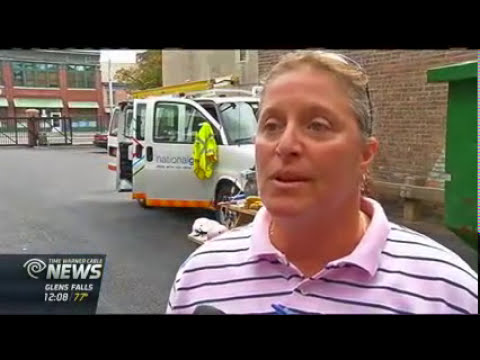The image is a screenshot from a Time Warner Cable News broadcast, identified by the logo and details in the bottom left corner, which shows "Glens Falls," "1208," and "77 degrees" against a navy blue background. The scene, set in an asphalt alleyway, features a woman of Caucasian descent with a strong jawline, deep-set eyes, and gray-streaked blonde hair pulled back. She has a pair of sunglasses perched on her head and wears a pink collared polo shirt with horizontal black stripes. She appears mid-interview, with a partially visible microphone near her chest. In the background, there is a white utility van with all its doors open, yellow ladders mounted on top, and a yellow construction jacket hanging from it. The scene also includes a large green dumpster positioned in front of a brown brick building. The top and bottom of the image are cropped with black rectangles, adding to the broadcast's framing.